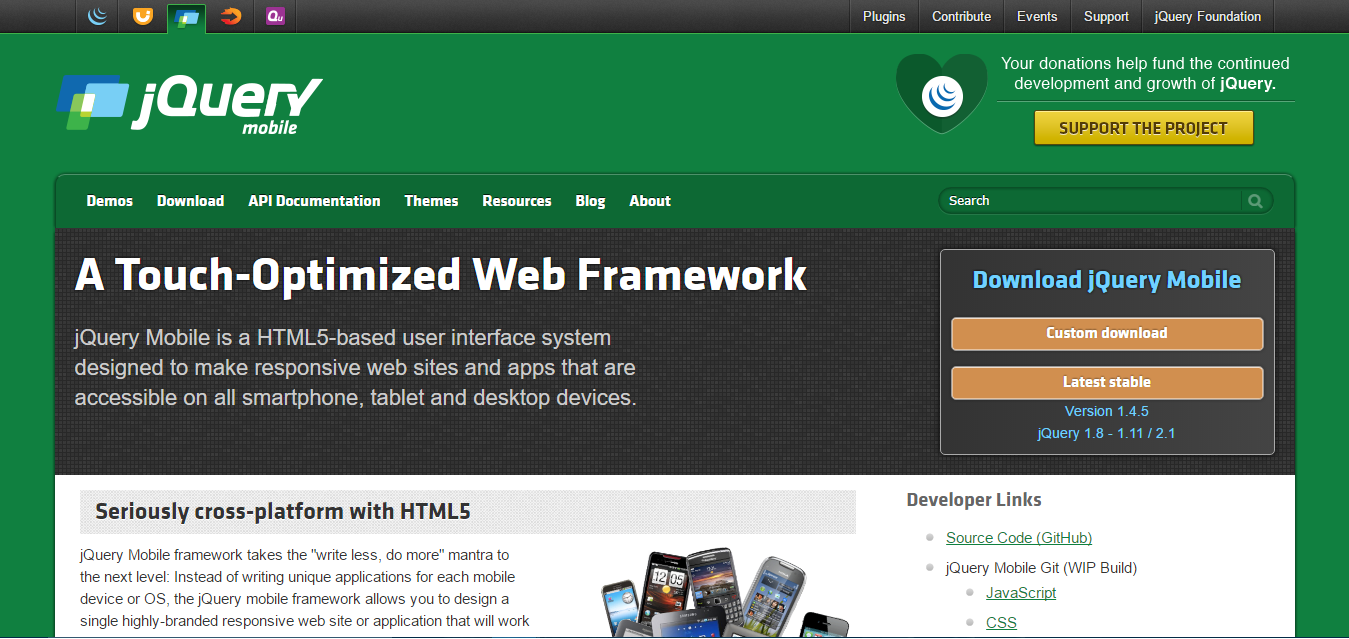The screenshot showcases a web page dedicated to jQuery Mobile. The background is a vibrant green, creating a striking visual contrast. At the top of the page is a black navigation bar containing five icons plus the words "Plugins," "Contribute," "Events," "Support," and "jQuery Foundation" aligned on the right-hand side.

Below the navigation bar, a bright green background dominates the screen. Centrally placed is the jQuery Mobile logo, consisting of a symbol with squares adjacent to the text "jQuery Mobile". On the right side of this logo is a darker green heart encircling a white circle filled with blue crescents. Accompanying this visual is the text: "Your donations help fund the continued development and growth of jQuery." Directly beneath is a yellow box with the phrase "Support the Project".

The next horizontal segment features another green bar listing the options: "Demos," "Download," "API Documentation," "Themes," "Resources," "Blog," and "About," with a search bar labeled "Search" on its right.

A black banner below this bar reads "A Touch-Optimized Web Framework" in white text. Underneath it, the description states: "jQuery Mobile is an HTML5-based user interface system designed to make responsive websites and apps that are accessible on all smartphones, tablets, and desktop devices."

To the side of this text is a blue square with the prompt "Download jQuery Mobile," followed by an orange box labeled "Custom Download." Further down, another orange box indicates "Latest Stable," with the text "Version 1.4.5 jQuery 1.8, 1.11, 2.1" beneath it.

At the bottom, a white box titled "Seriously Cross-Platform with HTML5" is displayed, featuring an image of multiple cell phones, highlighting the framework's compatibility with a range of devices.